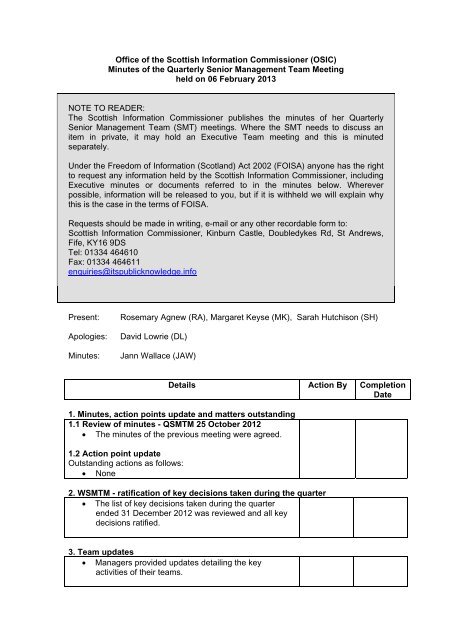This image is a scanned form from the Office of the Scottish Information Commissioner (OSIC) detailing the minutes of the quarterly senior management team (SMT) meeting held on 06 February 2013. The form has a white background with multiple lines of black text. At the top of the form, the title reads, "Office of the Scottish Information Commissioner (OSIC), Minutes of the Quarterly Senior Management Team Meeting Held on 06 February 2013." 

Directly beneath the title is a light-colored box containing a "Note to Reader," which explains that the Scottish Information Commissioner publishes the minutes of her quarterly SMT meetings. It also mentions that if the SMT needs to discuss an item privately, an executive team meeting will be held and minuted separately. The note further details that under the Freedom of Information (Scotland) Act 2002 (FOISA), anyone can request information held by the Scottish Information Commissioner, including the executive minutes or documents referenced in the minutes. Where information is withheld, an explanation will be provided in accordance with FOISA. Requests for information should be made in writing.

Further down, the form lists the attendees of the meeting: Rosemary Agnew, Margaret Keyes, and Sarah Hutchison were present, while David Launey gave apologies, and Jan Wallace took the minutes. Below this section, the form features a table with columns labeled "Details", "Action By", and "Completion Date". The table outlines three main points that need to be discussed:
1. Review of minutes, action points, update, and matters outstanding.
2. Ratification of key decisions taken during the quarter.
3. Team updates.

The detailed structure and procedural notes encapsulated in this form highlight the formal and comprehensive nature of the meetings and the importance of compliance with the FOISA.